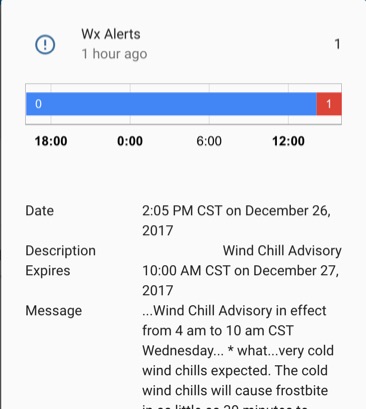Here's the cleaned-up, detailed caption for the image:

---

This image is a cropped screenshot of a weather information alert on a digital device. The layout features a light gray background with a thin black line running vertically along the left edge. At the top left corner, there is a blue exclamation point encircled in blue, next to bolded dark gray text reading "WXALERTS" where the "W" and "A" are capitalized. Below this text, there is a light gray timestamp saying "1 HOUR AGO."

In the top right corner of the screenshot, there's a black numeral "1". Directly beneath this number, a horizontal bar graph is displayed, which is approximately 90% blue extending from the left, and red for the remaining portion. On the left side of the blue section, there is a white numeral "0," while the center of the red section shows a white numeral "1."

Underneath the horizontal bar, there are bolded black times spaced evenly with corresponding vertical light gray lines intersecting the bar. The times listed from left to right are "1800," "0," "600," and "1200." 

Further down, the image is divided into two columns of information. The titles of these columns, displayed in black text, read "DATE," "DESCRIPTION," "EXPIRES," and "MESSAGE." 

The rows of information beneath these headers provide the following details:
- DATE: "2:00 PM CST on December 26, 2017"
- DESCRIPTION: "WIND CHILL ADVISORY"
- EXPIRES: "10 AM CST on December 27, 2017"
- MESSAGE: "...WIND CHILL ADVISORY IN EFFECT FROM 4 AM TO 10 AM CST WEDNESDAY. * WHAT... VERY COLD WIND CHILLS EXPECTED. THE COLD WIND CHILLS WILL CAUSE FROSTBITE."

The rest of the message is cut off at the bottom of the image.

---